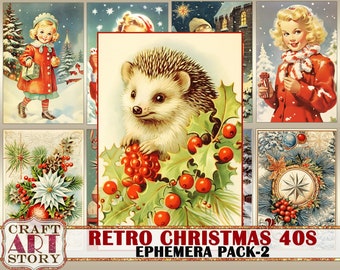This detailed image depicts a vintage-style Christmas poster titled "Craft Art Story," with the words "Retro Christmas 40s Ephemera Pack Two" highlighted at the bottom in red and black capital letters. Set against a background of eight images, four of which are obscured by a prominent central rectangle, the scene unfolds with charming holiday vignettes. 

In the top left corner, a young girl dressed in a red gown is seen walking through a snowy landscape, evoking a nostalgic winter wonderland. To the far right, another holiday image features a blonde girl in a similar red dress, adorned with a candy cane striped scarf, also standing in a snowy setting. 

On the bottom left, a delicate arrangement of white flowers, green leaves, and red berries decorates a serene white background, possibly mistletoe. The bottom right image showcases a circular ornament accented by red berries amidst a snowy backdrop, adding to the festive theme.

The centerpiece of the poster features a brownish hedgehog perched on a green surface, framed by more red berries, lending a whimsical touch to the overall design. The muted colors and intricate details throughout the images create a harmonious and nostalgic holiday aesthetic, encapsulating the charm of a Retro Christmas.